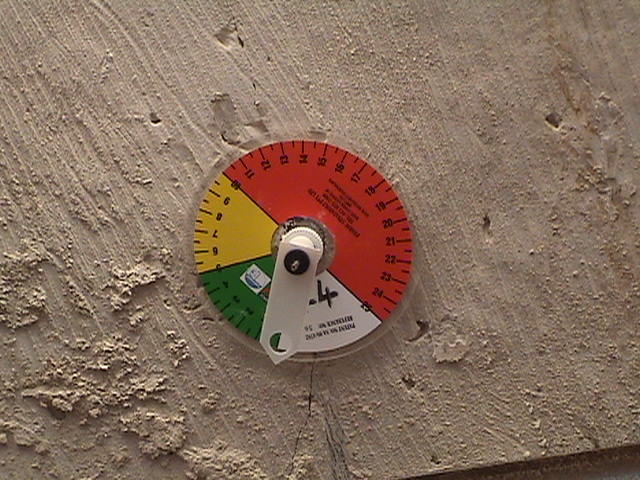The image features a highly textured wall with a predominantly clay or light brown hue, accentuated by distinct vertical lines. The left side of the wall is rougher with elevated areas and noticeable chips, lending it a dynamic, three-dimensional appearance. In contrast, the right side is smoother and more uniform.

Central to the wall is a circular object, cleverly designed and divided into four sections. One semicircle is vividly red and marked with numbers ranging from 10 to 25, each flanked by black lines, with additional black lines interspersed between the numbers. The other semicircle is trisected into three equal triangles colored yellow, green, and white. The yellow section is numbered from 5 to 10, while the green section is numbered from 1 to 4. The white section is left unnumbered.

In the center of this circular object is a white arrow-like piece, pointing between the green and white triangles. The white triangle contains text, as does the red section, distinguishing these areas with additional detail.